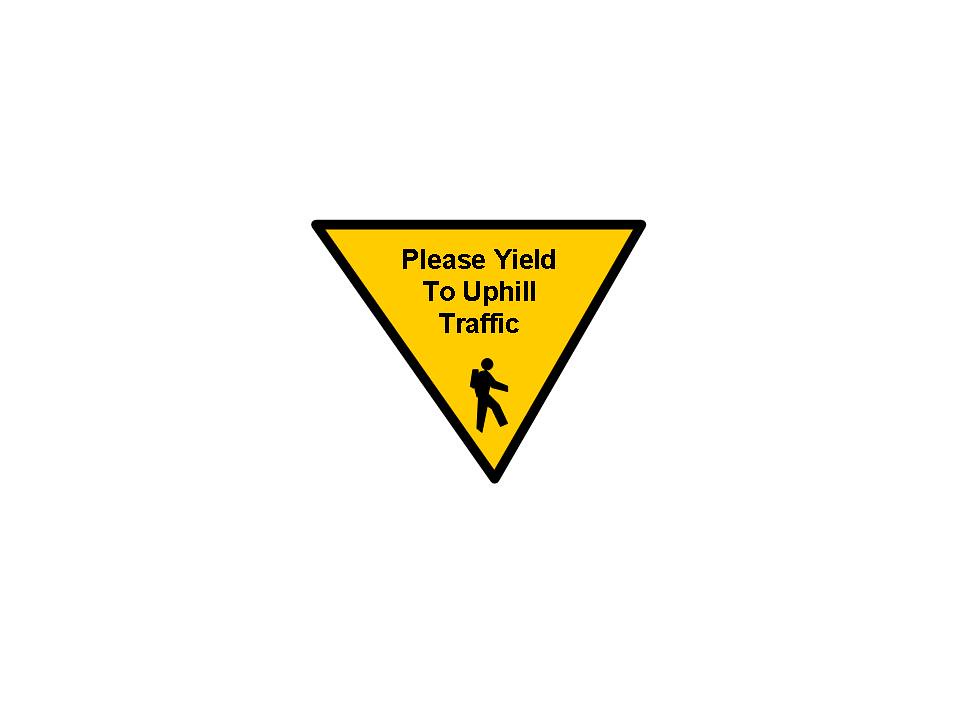This detailed description is based on an audio-recorded caption for an image:

The graphic in question depicts a yield sign in the shape of an upside-down triangle. The sign has a yellow background with a black border. At the top of the sign, there are black words that read "Please Yield to Uphill Traffic." Below the text, within the triangle, is the silhouette of a person. This figure features a round head, with legs apart as if in motion. The person’s arms are stretched out in front, and they are carrying a small square backpack on their back. The sign has no background elements, focusing solely on the yield sign and the walking figure at the bottom of the triangle.